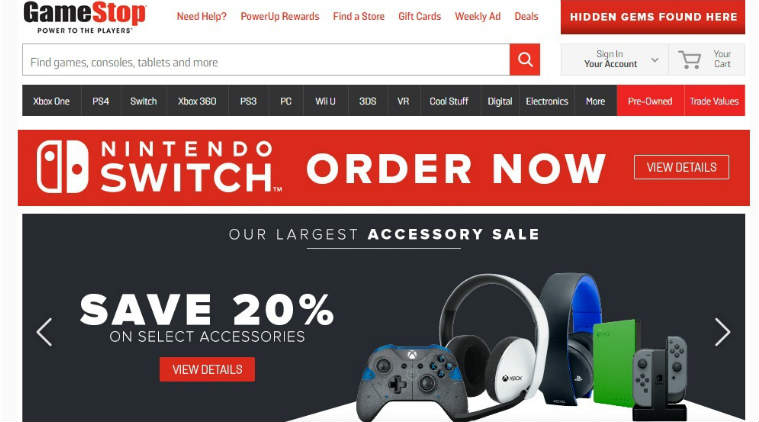The image showcases a computer screen displaying the GameStop website. Prominently featured at the top-left is the GameStop logo accompanied by their slogan, "Power to the Players." 

On the right side of the header are several navigation links: "Need Help?", "Power Up Rewards," "Find a Store," "Gift Card," "Weekly Ad," and "Deals." Adjacent to these links is a rectangular red box with white text that reads "Hidden Gems Found Here."

Directly below the navigation bar, there is a search bar with the placeholder text, "Find Games, Consoles, Tablets, and More," accompanied by a magnifying glass icon. Next to the search bar, there are icons for "Sign into your account" and a shopping cart.

Following this section, there is a horizontal menu listing various product categories: "Xbox One," "PS4," "Switch," "Xbox 360," "PS3," "PC," "Wii U," "3DS," "VR," "Cool Stuff," "Digital Electronics," "More," "Pre-Owned," and "Trade Values." Specific promotions are also highlighted, such as "Nintendo Switch," with options to "Order Now" and "View Details."

Further down the webpage, there is a black promotional banner advertising "Our Largest Accessories Sale," offering a 20% discount on select accessories, with a link to "View Details." To the right of this banner, images of gaming headsets, controllers, and speakers are displayed, emphasizing the accessories on sale.